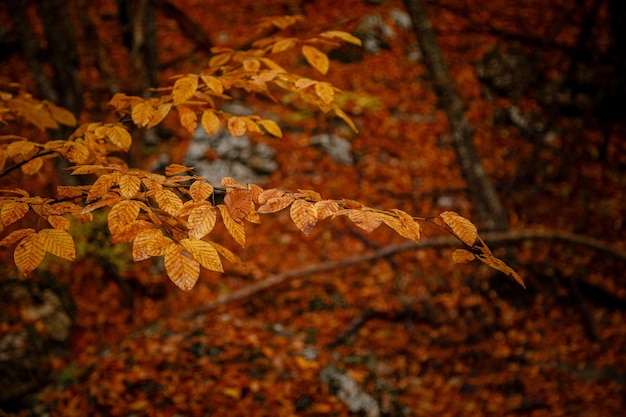This photograph captures a picturesque autumn scene within a forest. A branch stretches from the left side of the image into the foreground, adorned with golden amber leaves, each leaf’s veins clearly visible, accentuating the intricate details. Behind this branch, the background blurs into a tapestry of fallen leaves in various shades of red, orange, and yellow, painting the forest floor with vibrant autumnal hues. Scattered among the leaves are a few narrow, brown branches, while patches of gray ground occasionally peek through the dense leaf cover. The overall muted colors enhance the serene beauty of this fall landscape.